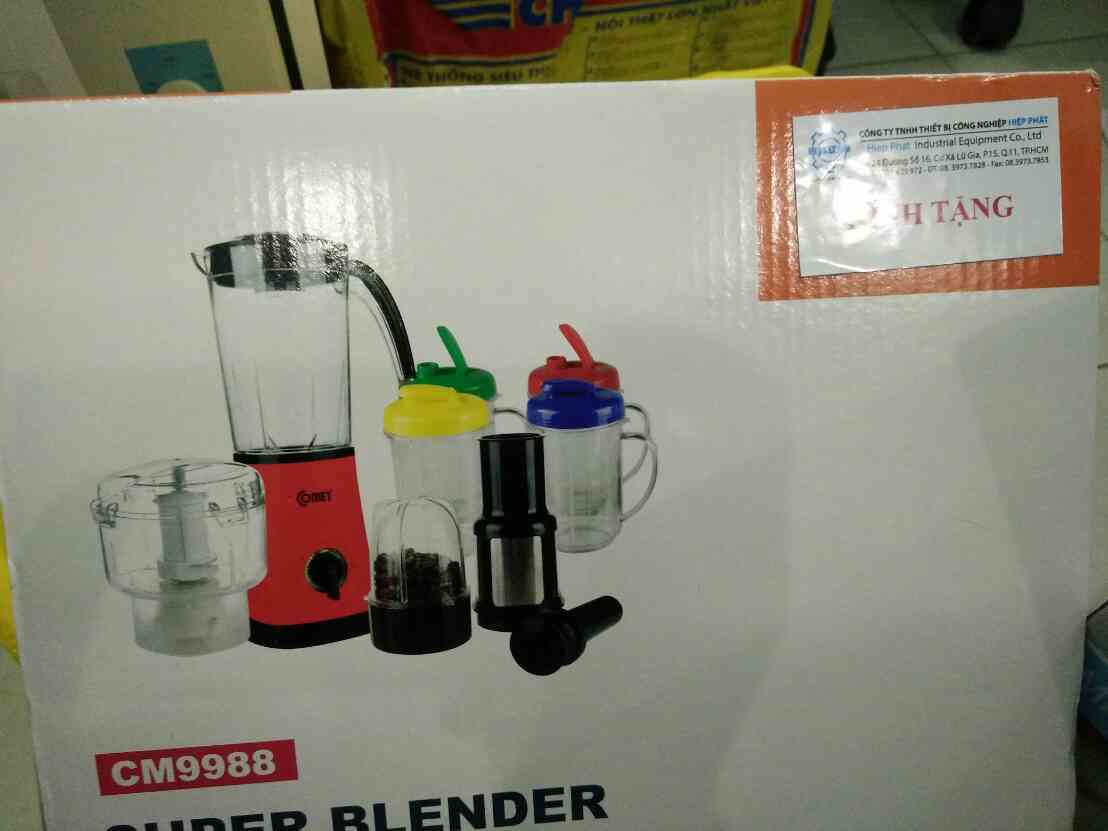The photograph depicts the front of a white cardboard box featuring a variety of kitchen appliances and accessories, prominently showcasing a red blender. The blender has a clear pitcher with a black handle and a black toggle switch on its base, which is also red. To the left of the blender is a circular food processor attachment with a clear lid and a long white center. Also visible is a small black half-cylinder attachment piece. Behind this setup are four clear cups or pitchers, each with a handle and a lid that comes in different colors: yellow, green, red, and blue, with spouts incorporated into the lids. Additionally, there is a black cylinder, likely a pusher tool for food processing. At the bottom of the image, written in white text inside a red rectangle, is the model number "CM9988" with the word "Blender" in black text below it. The brand name is partially obscured in the lower-left corner, and there are light reflections on the box that slightly obscure some details.